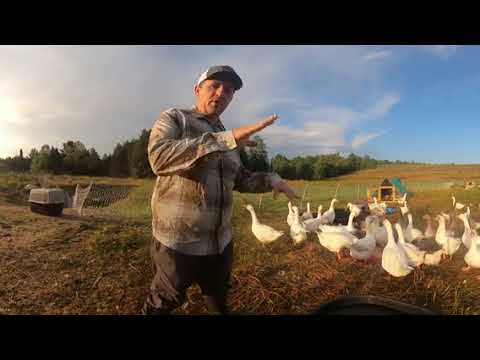In the photograph, taken outdoors on a spacious farm, a man stands at the center engaged in an animated discussion, his hands gesturing as if giving instructions. He is dressed in a tan and white plaid shirt, brown pants, and a ball cap. To his right, a considerable gathering of around 25 to 30 white geese or ducks are huddled together next to a water trough. Behind these birds, their housing structure, identifiable by its distinctive green metal roof, is visible. On the left side, there's a large cage with a brown bottom and a white top, accompanied by a somewhat dilapidated fence. The background is adorned with tall evergreen trees, and the foreground showcases a vast field with patches of grass, some of it appearing brown or dead. The setting is completed by a blue sky dotted with clouds, creating a serene farm-like atmosphere.